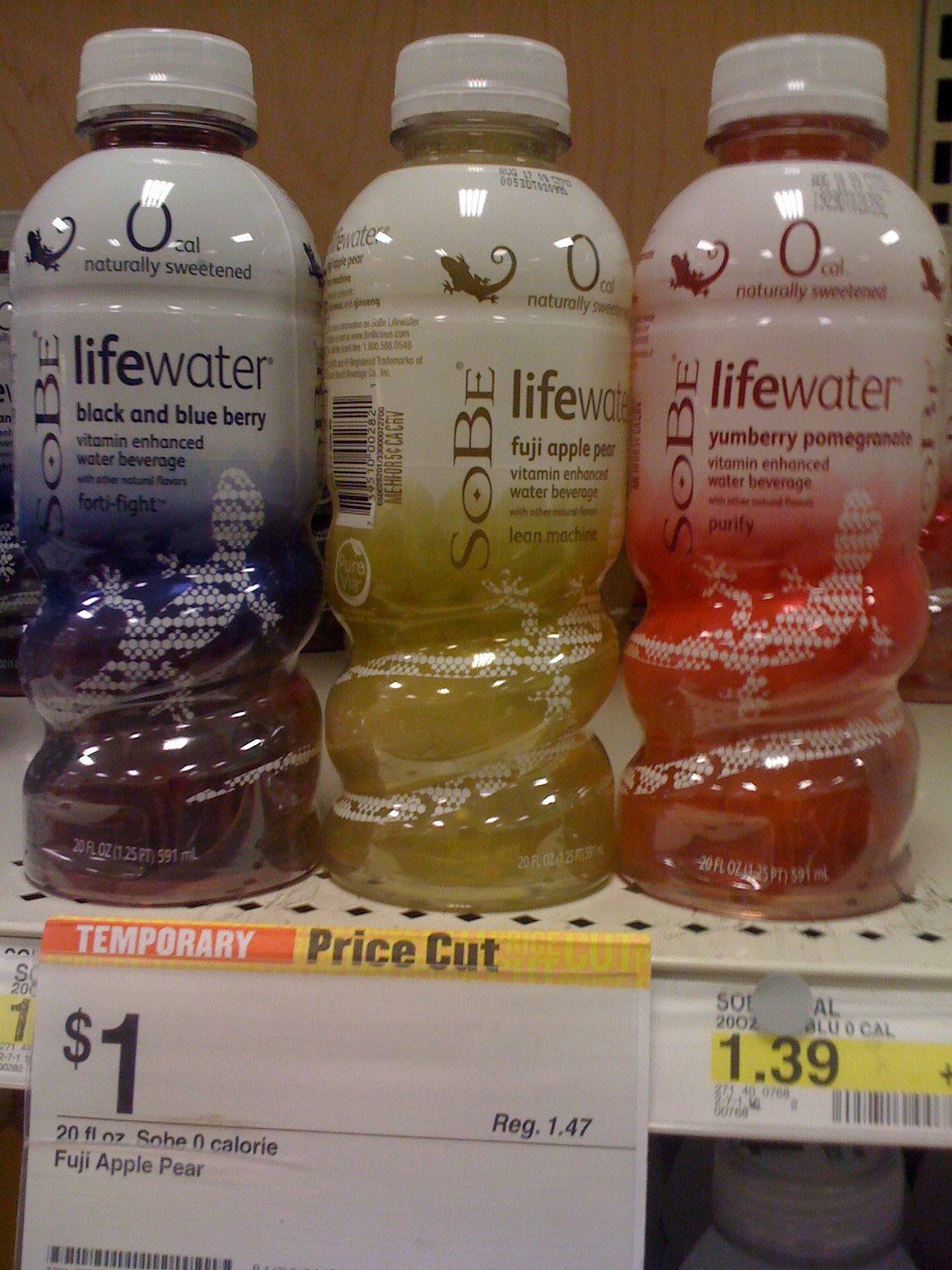The image depicts a scene from a Target store, featuring three bottles of Sobe Lifewater positioned on a top shelf, as no items are displayed above it. Each bottle is marked with the Sobe logo on the left side and the label "Lifewater" stretching across. The bottles are aligned left to right, with the flavors and color schemes as follows: the leftmost is black and blueberry with a blue and white label, the middle bottle is Fuji apple pear featuring a white and yellow label, and the rightmost is yum berry pomegranate with a white and red label. All three bottles have semi-transparent whitish caps and display a small gecko pattern symbolizing the company's logo.

The shelf holds a promotional sign that reads "Temporary Price Cut," indicating a reduced price of $1 from the original $1.39. An additional shelf tag reiterates the original price of $1.39, along with a visible QR code. Behind the bottles, the backdrop is a brown wall. Below the top shelf, part of a cap from another bottle is visible, hinting at another shelf beneath. The scene is meticulously organized, emphasizing the sale and arrangement of the Sobe Lifewater bottles.